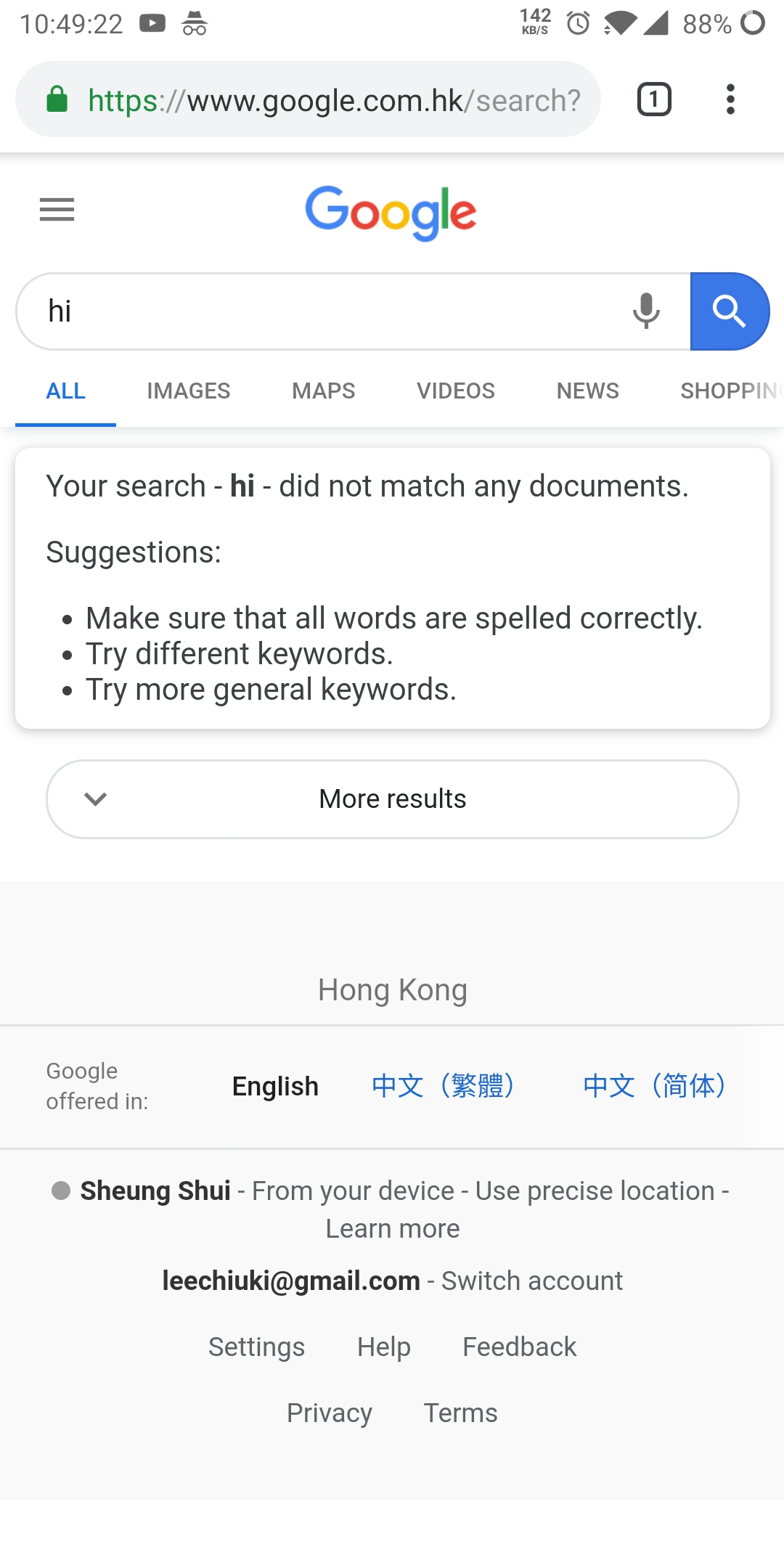A screenshot captured on a mobile device showing a Google search conducted using the term "high," which resulted in no matching documents. The Google search interface advises the user to ensure all words are spelled correctly, try different keywords, or use more general keywords. This search is conducted on the Hong Kong version of Google, accessible via https://www.google.com.hk, with the interface available in multiple languages including English, Traditional Chinese, and Simplified Chinese.

The screenshot also reveals detailed device information. The time displayed on the device is 10:49:22, the battery level is at 88%, and the Wi-Fi signal is strong. Additionally, there is a data usage indicator showing 142 kilobytes per second. The Google interface is in English, and the precise location of the device is in Shangshu. The search was performed using the Gmail account lee.ch.i.u.k.i@gmail.com.